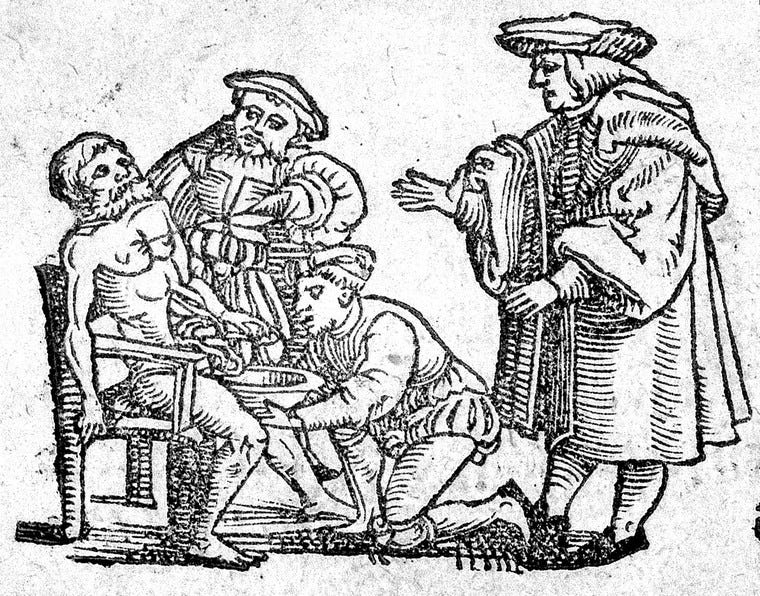This detailed black-and-white drawing from the Middle Ages, possibly from the 1300s or 1400s, depicts an early form of medical practice involving several figures. On the left side of the image, a sickly, largely naked man is sitting in a four-legged chair, with only a tunic around his waist. His head is tilted back in discomfort as he pulls his innards out, or so it appears. Kneeling to his right is a man in a jester outfit, holding a bowl beneath the patient's organs, possibly to catch them or assist in some manner. Another large-set, bearded man is touching the patient's chest with a stick, which might be intended to ward off evil spirits, as he gazes intently at the sick man. A fourth figure, wearing elaborate robes and a hat similar to the man holding the stick, stands nearby with one hand extended toward the patient, possibly in a gesture of offering prayer or directing the procedure. The detailed and somewhat eerie scene is entirely in black and white, capturing a grim yet intricate portrayal of medieval medical practices.